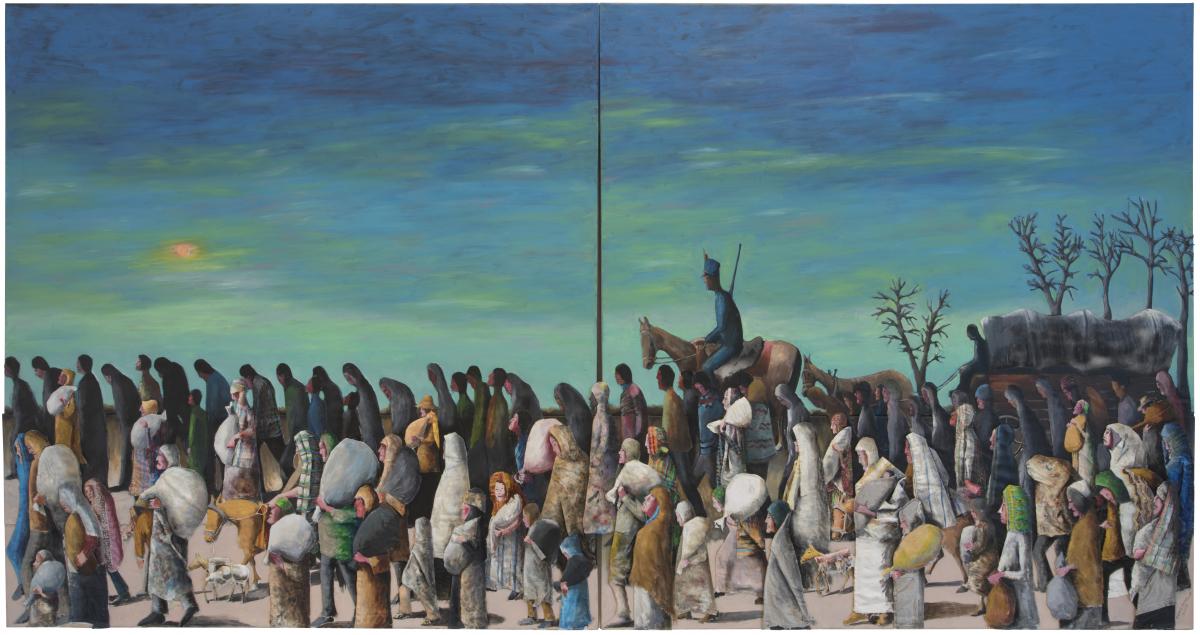This detailed painting, rendered in vibrant colors and historical style, portrays a somber scene of forced migration, likely depicting the displacement of the Cherokee people during the Great Migration. The painting is landscape-oriented and captures a large crowd of people, many of whom are wearing long, layered clothing and carrying bundles on their shoulders and under their arms. The people, depicted as Native Americans and peasants, are moving from the right to the left of the image. 

Towards the bottom of the image, numerous figures are arranged in different rows, emphasizing the scale of the march. A noteworthy feature is the rider on a horse positioned on the right side of the painting. This rider, dressed in a blue uniform and armed with a rifle, appears to be overseeing the march. Near the rider, there is a covered wagon being pulled by a horse, and behind the wagon, barren trees devoid of leaves are visible, marking the only area in the image with any form of natural landscape. 

The top half of the painting is dominated by a striking sky, which transitions from blue to green. On the left side of the sky, partially obscured by clouds, is a circular, orange area that suggests a setting sun, contributing to the melancholic atmosphere of the scene. Notably, a line down the center of the painting draws attention to a gruesome detail: what appears to be a young woman impaled on a stick, adding to the gravity and poignancy of the historical event being depicted.